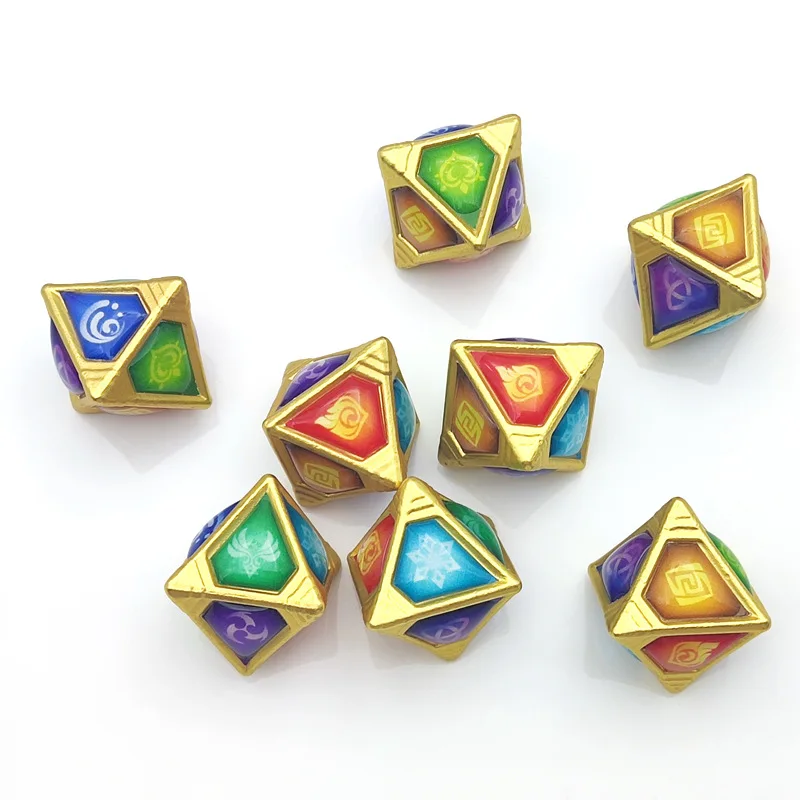The image depicts a collection of pyramid-shaped spinning toys, each adorned with triangular faces in a variety of vibrant colors. The toys feature approximately ten distinct sides, each side forming a triangle. The faces of the pyramids are painted in diverse hues, including blue, green, red, light blue, purple, and gold. The entire structure has a golden finish, creating an impression as if it was dipped in gold, with the colorful triangular facets adding a striking contrast.